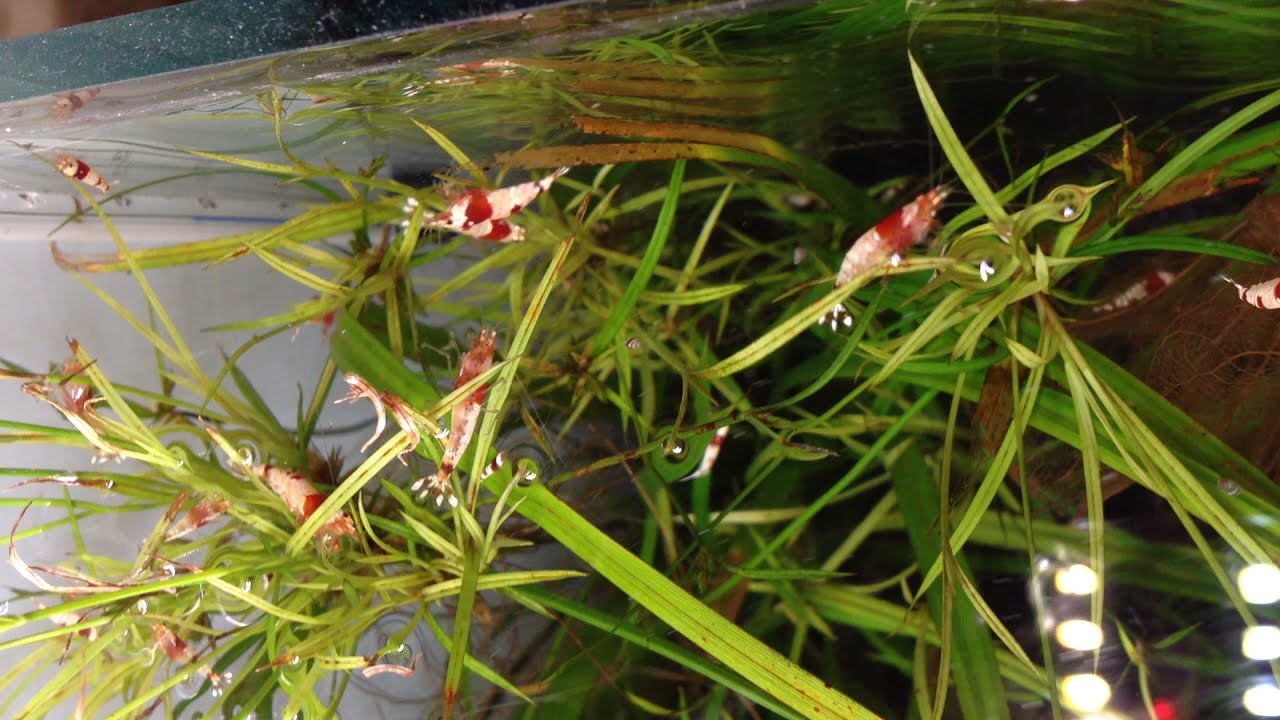This image showcases the interior of a small aquarium taken from a downward angle. The tank is filled with abundant grass-like vegetation, characterized by long, thin, green leaves that resemble blades of grass. Tiny air bubbles are visible on the surface of the leaves, glistening in the light. Amongst the vegetation, dozens of distinct, brightly colored shrimp are congregated. These shrimp feature striking red stripes along their white bodies, giving them a unique, eye-catching appearance. In the background, the aquarium's gray, possibly metallic ceiling is discernible. Near the lower right-hand corner, six glowing white orbs of light are reflected off the water's surface, with a mirror situated between some of the lights. The image also captures the edge of the tank in the upper left-hand corner, which appears black and slightly dusty. The detailed arrangement of flora and fauna combined with the lighting creates an engaging and serene aquatic scene.